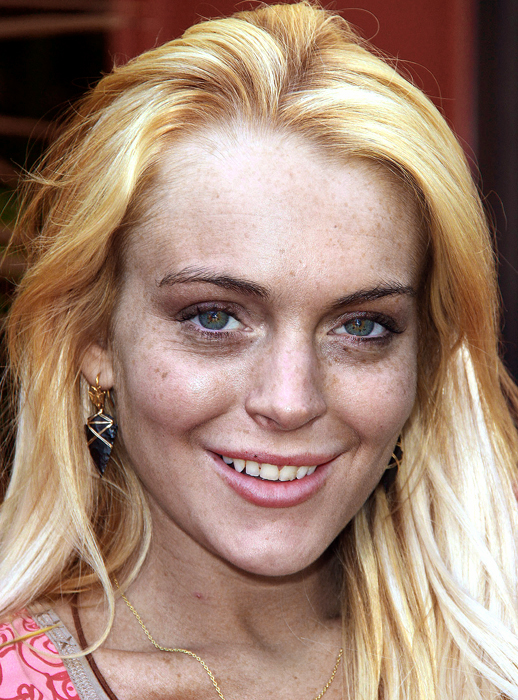This image is a close-up of Lindsay Lohan, who is looking directly at the camera with a smile, revealing her upper set of teeth. Her long, straw-yellow blonde hair drapes over her right shoulder. She has a fair complexion adorned with freckles on her face, particularly across her forehead and cheeks, and she has hazel or greenish eyes. Her eyebrows are brown, and she has noticeable lines under her eyes, adding a touch of age to her appearance. She is wearing a thin gold chain necklace and black arrowhead-shaped earrings with gold and dark blue accents. Although the pink shirt she is wearing is mostly hidden, a hint of it is visible in the lower left corner of the image. The background is blurry, with indistinct patches of white, black, and red colors. Additionally, there appears to be a small piece of pepper between her teeth.